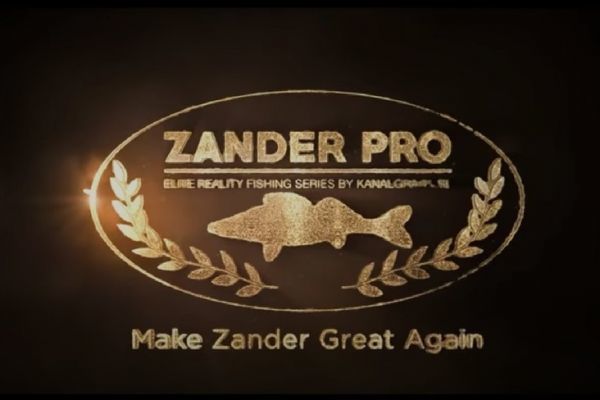The image features a landscape-oriented emblem with a predominantly dark brown to black background. Centered is a prominent horizontal gold oval with intricate decorations. At the top of the oval, in bold, uppercase gold letters, is the text "Zander Pro," underlined by a bar. Below this, in smaller but still gold uppercase letters, it reads "Elite Realty Fishing Series by Canal." The central part of the emblem showcases the gold outline of a fish, flanked by two golden leaves on either side. Toward the bottom of the oval, in the same gold font and style but in lowercase, is the phrase "Make Zander Great Again." The left side of the emblem is softly illuminated by a bright light, creating a subtle transition to a brownish hue. This emblem likely represents a logo for a fishing company or a related series, emphasizing gold lettering and detailed ornamental design set against the dark background.